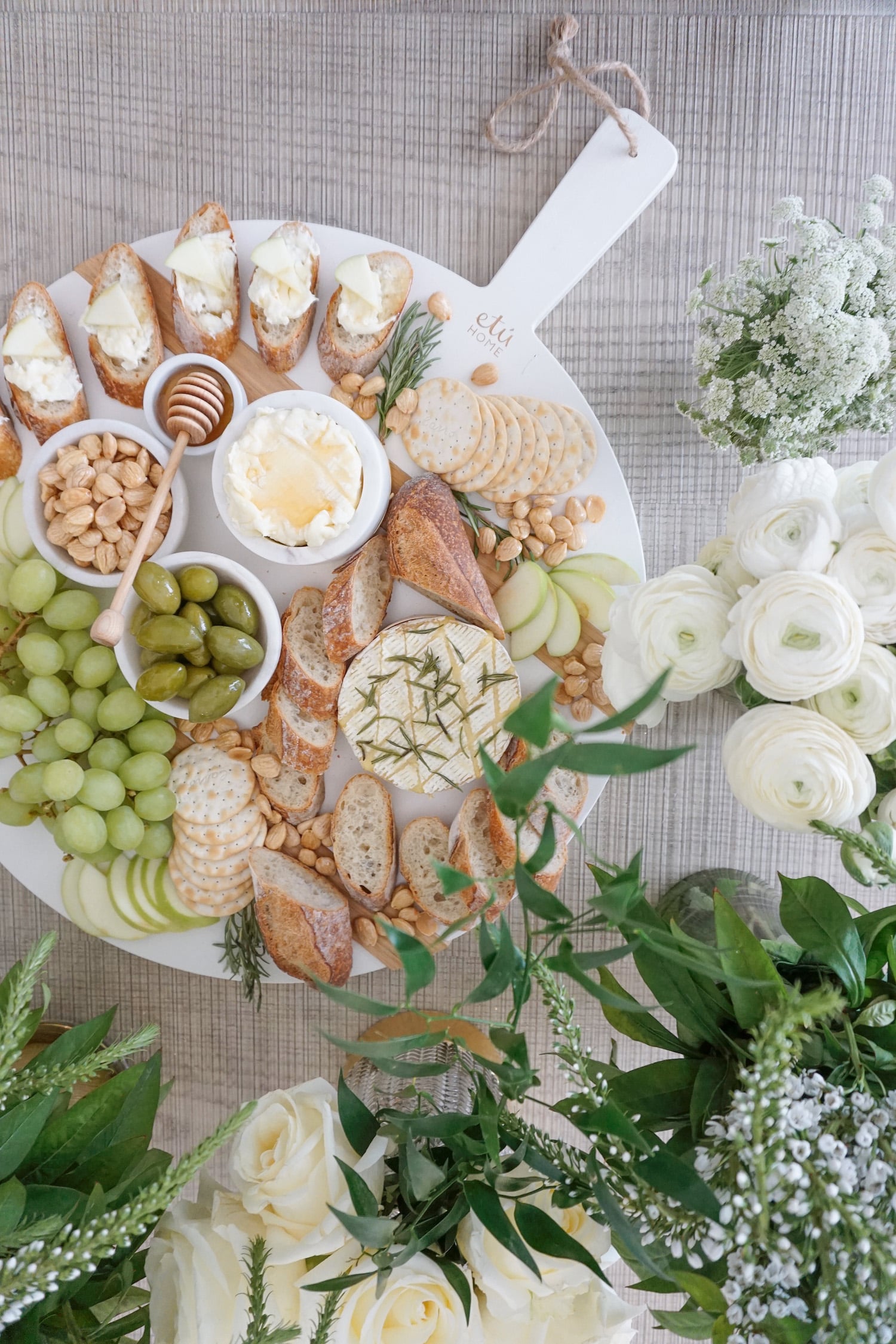This vibrant overhead image captures a meticulously arranged charcuterie board set on a light wooden table adorned with white roses, baby's breath, and lush greenery. The charcuterie board features a white circular plate with a handle extending to the top right. Around the edge of the plate are neatly arranged slices of baguette, some of which are topped with a creamy white cheese. In the 1 o'clock position, several water crackers are placed next to a collection of light brown nuts and bright green apple slices. Below these are more baguette slices followed by additional table crackers spanning from the 6-7 o'clock position. Bright green grapes occupy the 7-9 o'clock section of the plate. The center of the plate hosts an assortment of olives, a small amber pot of honey, a bowl of goat cheese drizzled with honey, and a honey stirrer. Scattered thoughtfully among the items are more grapes, crackers, brie, and nuts. The entire arrangement is framed with a stunning display of white roses and dark green foliage, creating an elegant and inviting presentation.